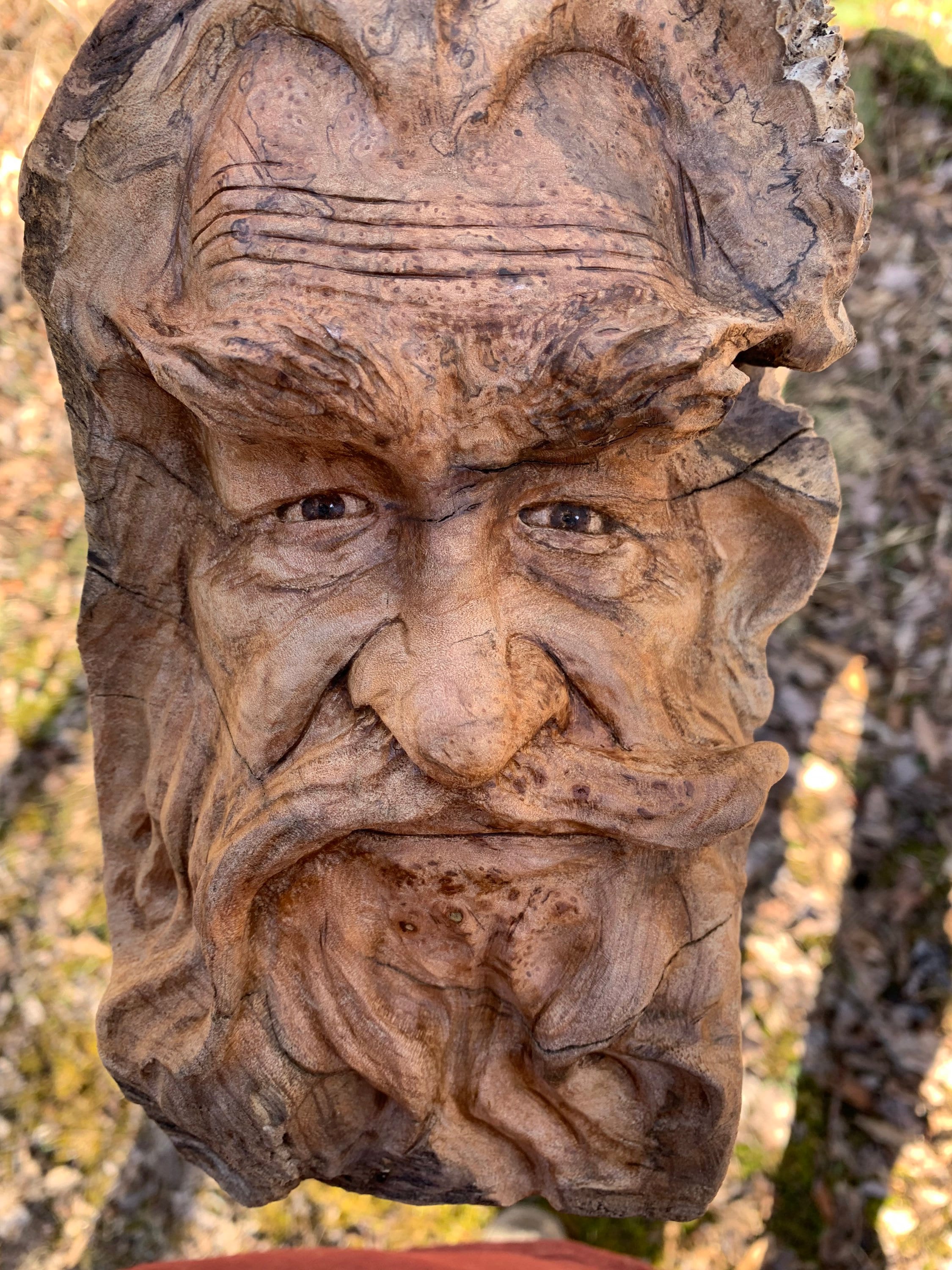This photograph captures a highly detailed three-dimensional carving of an old man's face, sculpted from a tree trunk. The man's face, possibly resembling the wizard Gandalf from Lord of the Rings, features prominent bushy eyebrows, a deeply furrowed brow, a long nose, squinting dark eyes, and a flowing beard and mustache. His hair, seamlessly blending with the tree bark, cascades down the sides of his face. The carving, tinted in various shades of brown and tan with some black accents, stands out vividly against a daytime backdrop adorned with vibrant fall foliage in hues of orange, red, yellow, and green. Shadows cast by the sun enhance the texture of both the carving and the surrounding leaves scattered on the ground. The photograph, taken from an elevated angle and looking downward, lacks any human figure for scale but suggests the work of a professional artist. Though not a professional photograph, it clearly showcases the intricate craftsmanship of the tree carving. A small red spot beneath the sculpture adds a mysterious element to the composition.